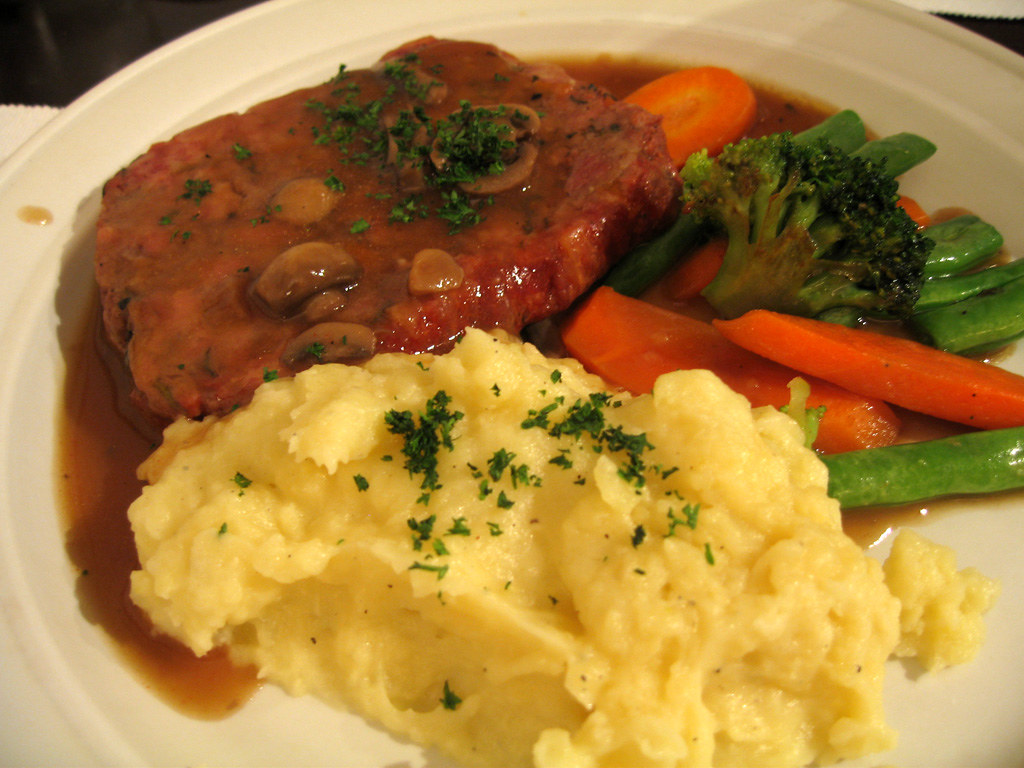The image features a white plate filled with a well-arranged meal. Dominating the lower portion of the plate is a generously served portion of mashed potatoes, slightly yellowish and sprinkled with small pieces of parsley. Above the mashed potatoes sits a large piece of meat, possibly meatloaf, lavishly covered in rich, brown gravy that spills over slightly, mingling with the other elements of the dish. On top of the meat, there are visible mushrooms and additional parsley pieces, adding to the garnish. On the upper right section of the plate, a medley of vegetables can be seen, including three pieces of carrot, several green beans, and a single piece of broccoli. The food items are starting to blend together due to the gravy, creating a cohesive and appetizing look. The white plate is partially visible around the edges, though not entirely shown, and the background features a contrasting mix of white and black colors.